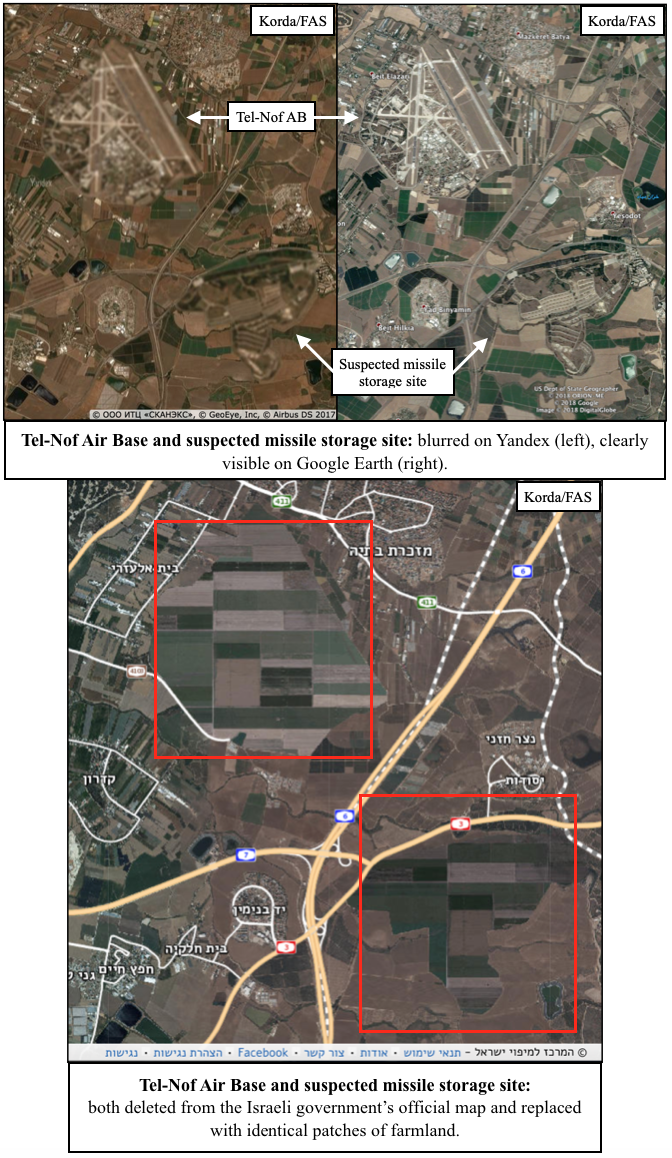The image comprises three aerial views with accompanying textual details, highlighting a suspected missile storage site at Tel Nof Air Base. The top-left portion of the image features an overhead shot primarily displaying brown soil interspersed with patches of green grass. Below this, bold text identifies the location as "Tel Nof Air Base and Suspected Missile Storage Site." Various arrows overlay the image, pointing towards grassy areas surrounding the suspected missile storage site within the town's vicinity.

The second section of the image zooms further into these rural zones, where hues of black, brown, and green dominate the landscape, depicting the farmland. A red square outline marks the upper left and bottom right corners, indicating the precise location of the suspected storage site. This section is effectively represented in an official map released by the Israeli government, detailing identical farmland patches that match the real photos above.

Overall, the image intricately combines satellite imagery and maps to pinpoint and label the Tel Nof Air Base and the associated suspected missile storage site, creating a comprehensive visual assessment of the area purportedly used for missile storage.